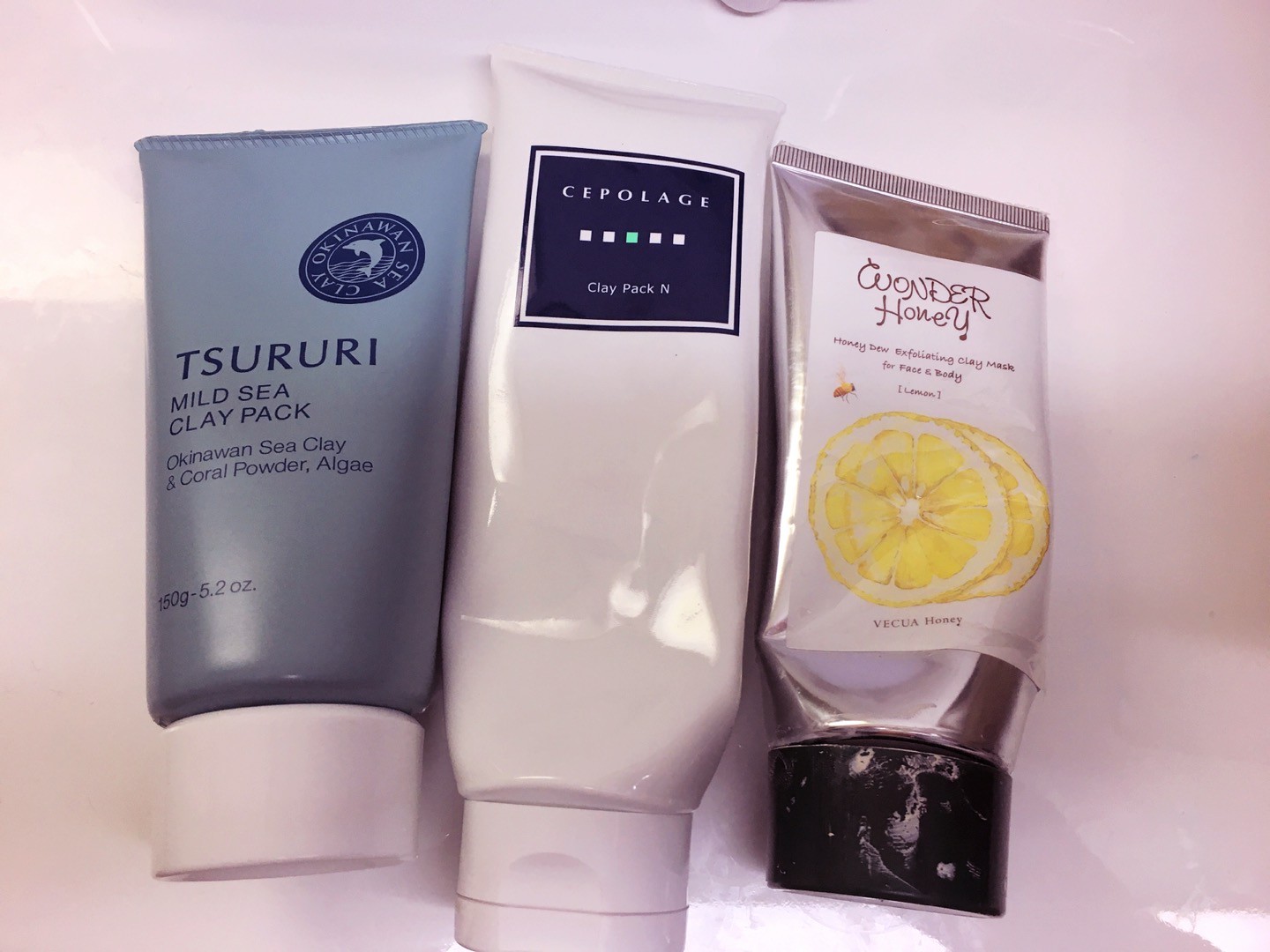In the image, there are three tubes of beauty products: Sururi Mild C. Clay Pack, Cepelage Clay Pack, and Wonder Honey. The Sururi Mild C. Clay Pack on the left features sleek silvery blue packaging with a white lid. The brand name "Sururi" is printed in navy blue, and above it, there’s a white circle containing white writing and an illustration of a dolphin. The tube also indicates its size: 150 grams / 5.2 ounces.

The middle product, Cepelage Clay Pack, is housed in a distinct, minimalistic tube. At the top, "Cepelage" is written in white against a black background, followed by five small white squares in a row. Below this, "Clay Pack" is printed in a clean, straightforward font.

On the right, the Wonder Honey tube stands out with its striking silver design. It features a white label, which occupies the entire bottom half, adorned with the realistic imagery of two lemon slices. The harmonious blend of simple color palettes and citrus graphics creates an inviting appearance.